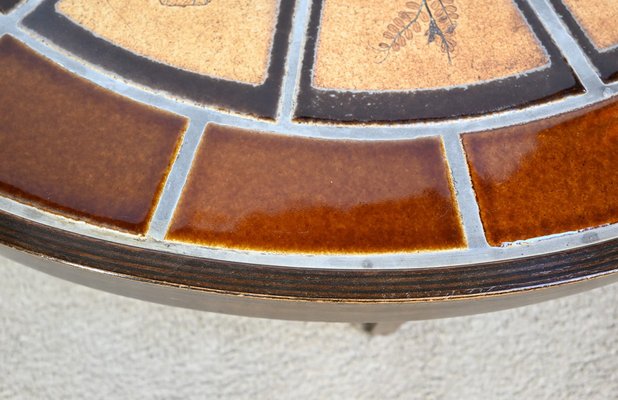The image features a detailed close-up of a ceramic plate with a glossy finish, taking up about three-fourths of the frame. The plate appears to be resting on a white, slightly textured surface, perhaps a cloth. Surrounding the plate is a dark brown or charcoal-colored rim that contrasts with the sections of the plate adorned with a mosaic-like design. This design includes three golden brown tiles set in a triangular pattern, light brown and tan tiles featuring a delicate plant stencil, and interspersed dark brown and black tiles. The intricate mosaic is framed by silver or steel pieces, giving the whole composition a rich and varied texture. The spaces between the tiles are filled with very light gray grout, enhancing the detailed arrangement.